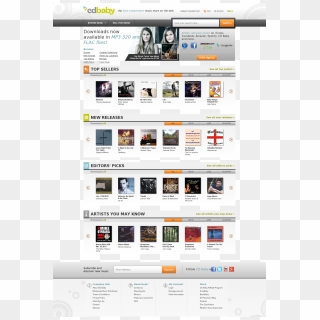This image showcases a highly blurred and small website interface, set against a gray and white checkerboard background. The central section of the image contains indistinct text, making it difficult to decipher any specific details. 

In the top left corner, there's a gray "C" and "D" with the word "baby" written in green nearby. Moving to the right, there are additional, indiscernible characters spread across a gray bar extending about an inch from both the left and right edges of the image.

Roughly two inches into the image, white letters appear both above and to the right of a white search bar with an orange tab. This text is also not legible due to the blurriness. Below this section, a highly unclear photo of two women is visible, with their faces being indistinguishable. To the left and right of this photo, there is some additional, unreadable information.

Further down, the text "Top Sellers" is somewhat discernible, listed above six indistinct images that could be album covers or books. Following this section, "New Releases" is similarly displayed with six more unrecognizable images beneath it. "Editor's Picks" continues the pattern with another set of six images, and finally, "Matches You May Know" is listed with another six images.

The lower part of the image features a second search bar with an orange tab to its right, followed by Facebook and Twitter icons, ending with more indeterminate text.